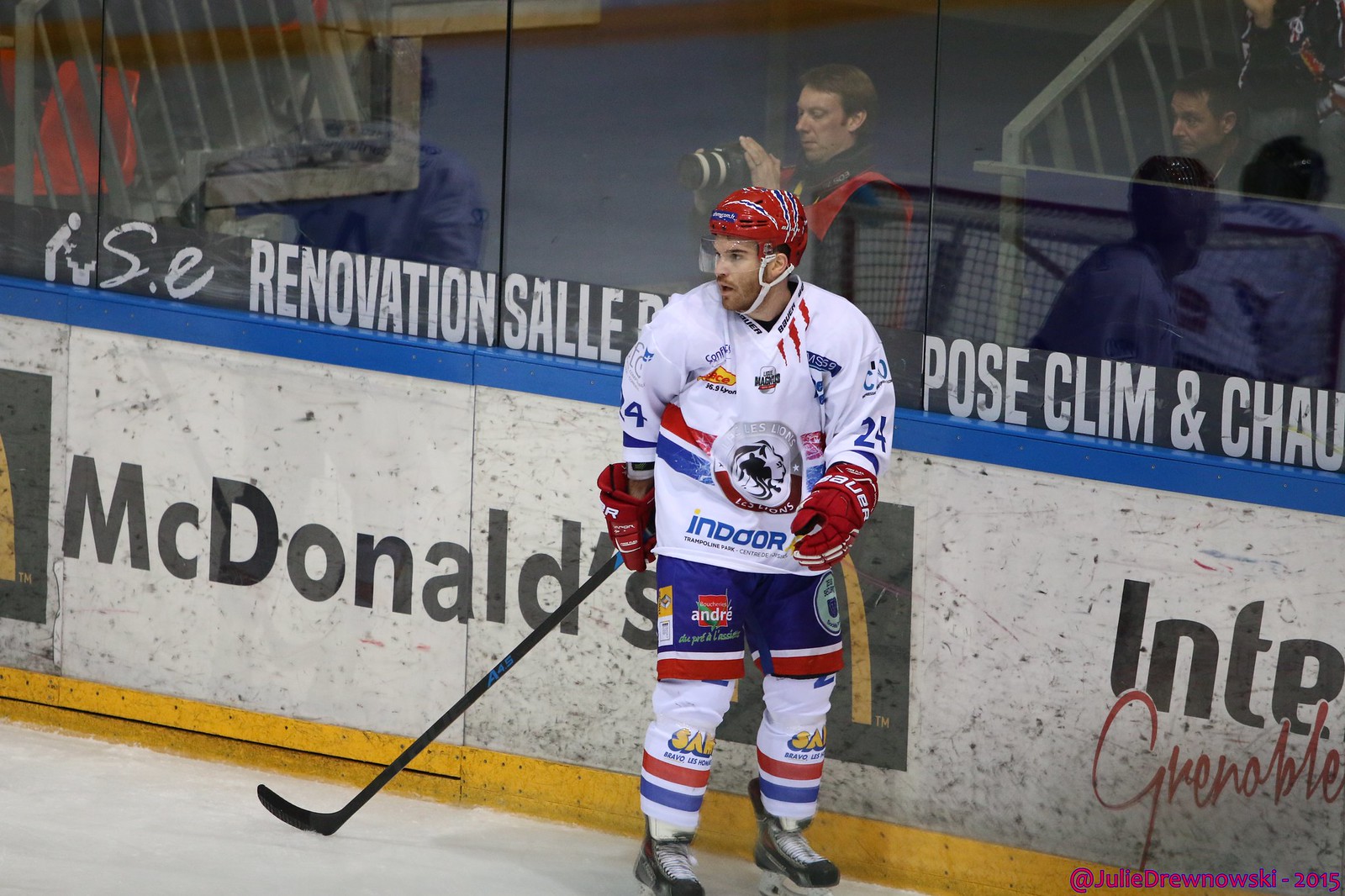The image depicts an ice hockey player captured indoors in a rectangular arena, wider than it is tall. The player, donned in a white jersey with blue shorts featuring red and blue trim and red gloves, stands on the ice rink. He’s sporting a red helmet and holding a black hockey stick in his right hand, while ice skates adorn his feet. His white pants peek out from beneath the shorts, completing the uniform detailed with a lion insignia on his chest encircled by a silver ring, reading "something lions" atop and "L-E-S lions" at the bottom. 

The arena’s environment features a white, blue-trimmed, yellow-bottomed safety wall behind the player, displaying advertisements including "McDonald's" and words like "renovation S-A-L-L-E" and "pose C-L-I-M and C-H-A-U." The upper section of the wall is made of plexiglass, through which a photographer in a red vest is visible, aiming his camera. Reflections of the audience and the stands can be seen on the glass, adding depth to the bustling atmosphere of the rink. The player looks to his right, seemingly in anticipation of the next move on the pristine white ice.